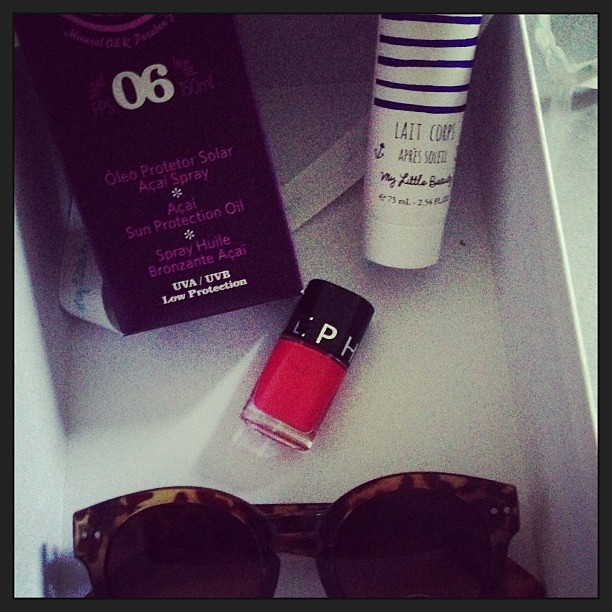In the photograph, a white rectangular container holds a collection of various personal care items, all enclosed within a black-framed image. At the bottom of the container, there is a pair of sunglasses with a leopard-print rim. In the center, a small jar of dark pink or red nail polish with a black lid sits prominently, bearing the letters LPH. On the upper left side, a rectangular case with text is visible; it prominently features the number "06" in white, and a description in purple or pink reading "Oleo Protector Solar Akai Spray," followed by "Akai Sun Protection Oil Spray Julil Bronzante Akai" and "UVA/UVB Low Protection" at the bottom. To the upper right is a white tube of cream or lotion with horizontal blue stripes across the top. This tube displays the text "Lait Corps Apres Soleil," meaning "Body Milk After Sun," and cursive writing below that says "My Little Beauty." The items are arranged within the container, which has raised sides, and a white ribbon with some blue writing, whose text is unclear, lies behind the items.